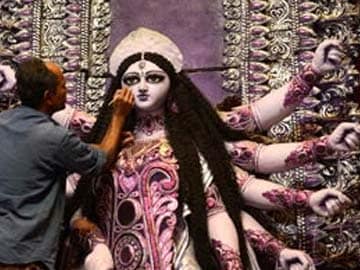The image depicts a balding man with a blue shirt, sleeves rolled up to his elbows, and brown skin, painting a statue of an Indian goddess. The goddess has long black cornrowed braided hair and features multiple arms, with five visible on her left side and the rest implied to be on her right side, partially obscured by the man. Her face is painted purplish-white with exaggerated features and large black eye shadow. A unique symbol, a line with a circle, is centered on her forehead. She wears a white tiara and a pink and black dress adorned with intricate swirly floral patterns, alongside a black and white circle resembling a Mayan calendar. The background is a purple wall with gold accents and a white lace-like ornate design. The image has a slightly grainy quality, making finer details less discernible.